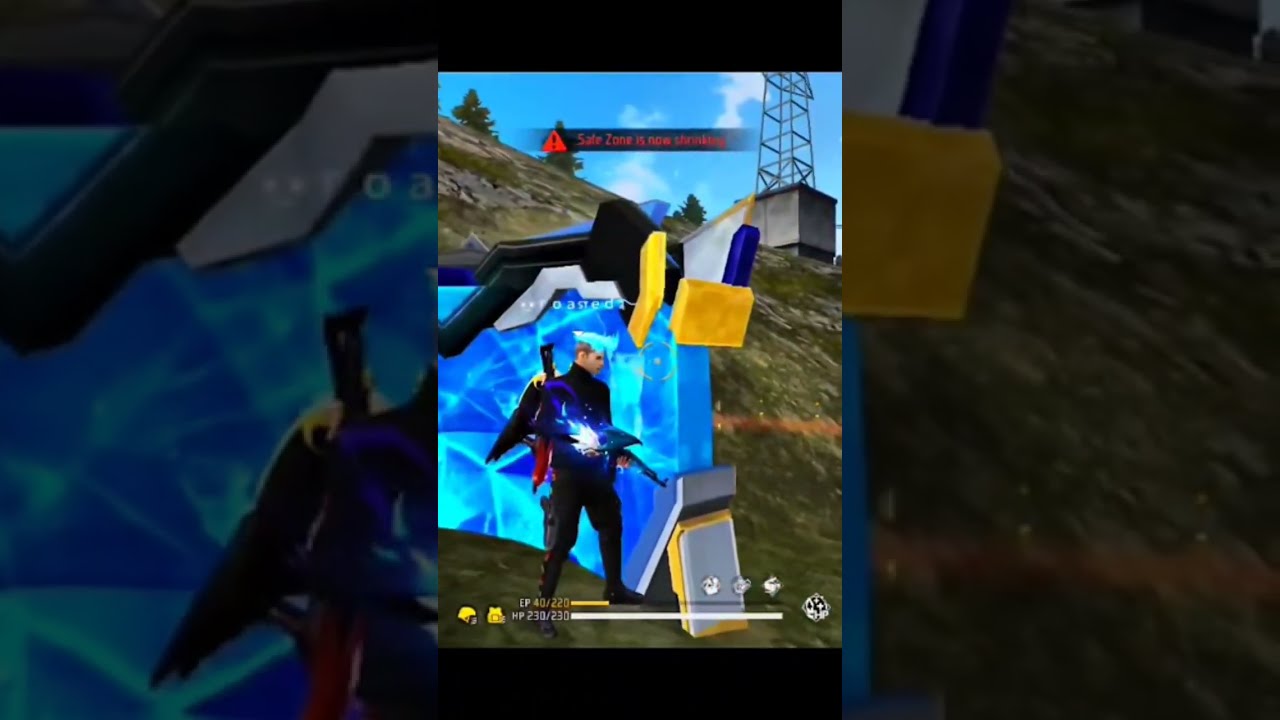In this screenshot from a video game, a male character clad in black pants and a black long-sleeve shirt stands prominently with a rifle pointed down towards his right. A bright flash of light is emanating from his stomach area. He is situated in front of a blue wall that appears to be made of glowing and dark blue hues, giving it an electric, field-like appearance. Behind this wall, a hillside slopes steeply downwards, topped with three trees. The sky above is a light blue with scattered clouds, contributing to the outdoor setting.

Additionally, there is a gray banner with a red triangle containing an exclamation mark and the text "safety zone" to its right. To the left of this banner, a radio tower rises into the sky with a gray box at its base. The landscape features patches of green grass mingled with light and dark brown soil.

At the bottom of the image, two level indicators are visible. The top indicator is yellow and shows about 10-25% fullness, while the line beneath it is white and extends completely across, indicating it is full. Menu icons or similar indicators are faintly visible in the bottom portion. The left and right sections of the screen are zoomed-in views of the background and the main character respectively, with both sections grayed out to about 50% brightness.